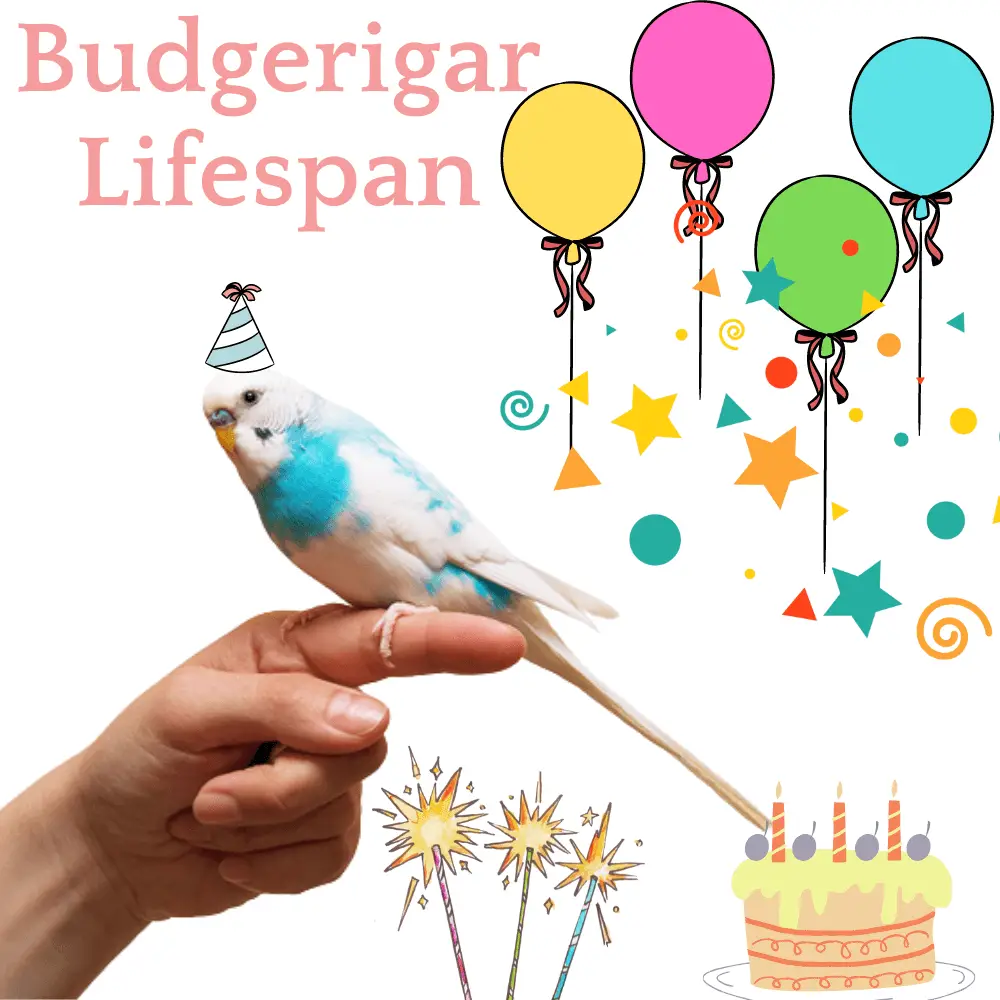The image is a combination of a photograph and graphic illustrations. In the bottom left corner, there is a realistic photograph of a white hand, likely a woman's, with the forefinger extended, upon which a blue and white budgerigar is perched. The bird, resembling a serene sky with clouds, sports a blue and white diagonally striped party hat with a little pink (or peachy orange) feather at the top, gazing leftward in a side profile showing one eye and a small yellow area near its beak.

The rest of the image is a montage of clip art. In the top left corner, "B-U-D-G-E-R-I-G-A-R" is written in pink letters with "lifespan" below it. Adjacent to this on the right, the top right corner showcases four festive balloons—yellow, pink, green, and blue—each with matching orange ribbons and strings. Scattered around the balloons are confetti graphics including stars, circles, and spirals in teal, yellow, red, and orange.

In the bottom right corner sits a clip art birthday cake, a light peachy orange color with alternating stripes and spirals, crowned with three red and white candles and four little purple decorations, possibly depicting fruit. Adjacent to the cake are three colorful sparklers—pink, yellowish-green, and blue—adding to the celebratory theme. The entire scene is set against a plain white background, combining real-life and whimsical graphical elements into a festive, vivid composition.